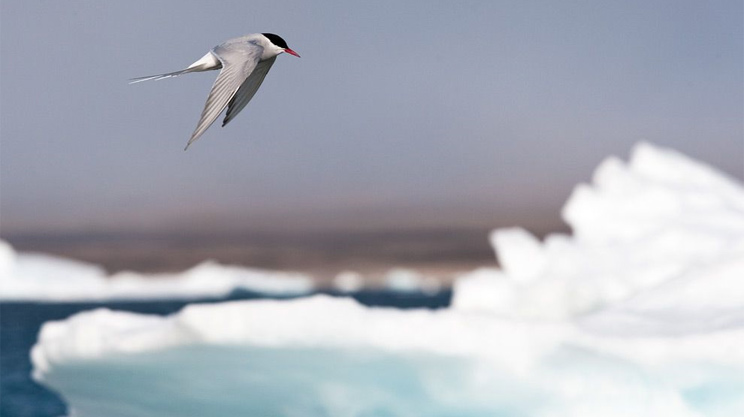In the photograph, a bird is captured mid-flight against a snowy landscape. The bird, with a white body, gray wings, and a relatively long gray tail, stands out with its black head and bright orange or red beak. Its wings are angled downward, indicating a recent downward wing movement. The background, though blurred, reveals a snowy terrain interspersed with patches of blue, likely a body of water. Snow blankets the bottom right and stretches across the image, with more snow visible in the distance. The background transitions into brown shades, hinting at land or dirt under the snow, and the sky above has a muted grayish-blue hue. The bird is flying towards the right side of the image, majestically navigating the wintry scene.